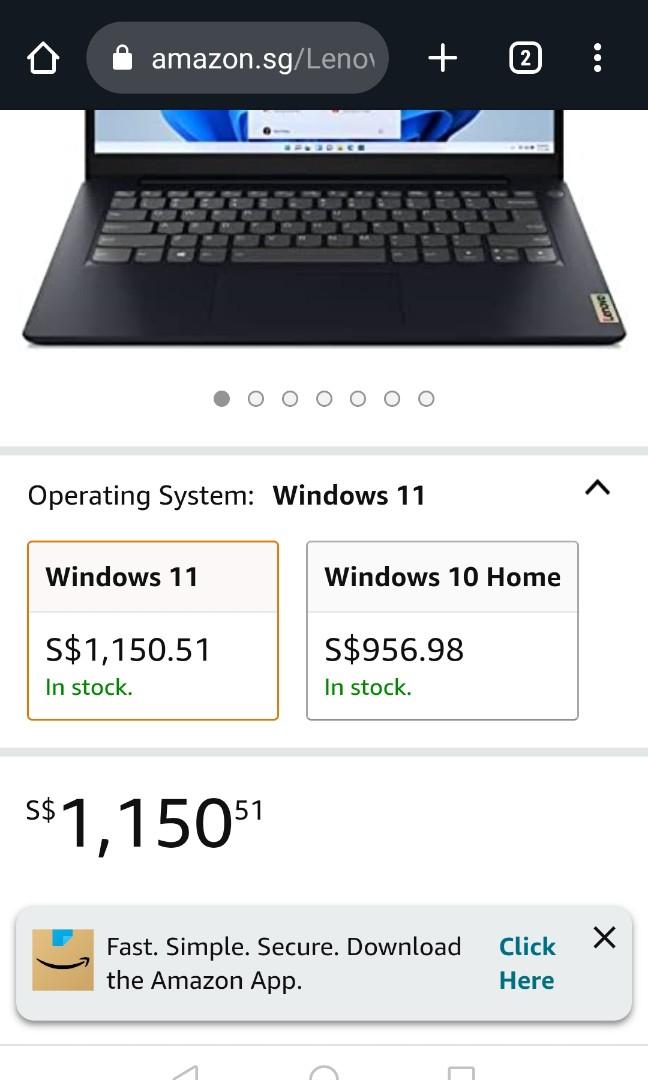This screenshot captures a product page on Amazon's mobile site, displaying a listing for a Lenovo laptop. At the very top, a black border indicates it's from a browser, and the partial URL "amazon.sg/leno" confirms the retailer and partial brand name. 

The main content features a close-up view of the laptop, focusing primarily on the keyboard area, which is medium gray against a dark gray, almost black, laptop surface. Just the bottom edge of the screen is visible, showing a faint light blue background with indistinguishable objects on either side of a white central element. 

Directly below the laptop image, a thin horizontal gray line separates the hardware details from a section listing the operating system options and their prices: Windows 11 priced at $1150.51, and Windows 10 Home at $956.98. Notably, the currency symbol used is 'S', though the specific currency is not indicated.

A secondary horizontal gray line follows, highlighting the Windows 11 option price in larger black font. At the page's bottom, a light gray rectangle with rounded corners promotes downloading the Amazon app, featuring the text "Fast, simple, secure." Next to this, a tan-colored square displays the Amazon smile logo, while blue text reading "click here" appears on the right side. A black X in the upper-right corner of this rectangle provides an option to close the box.